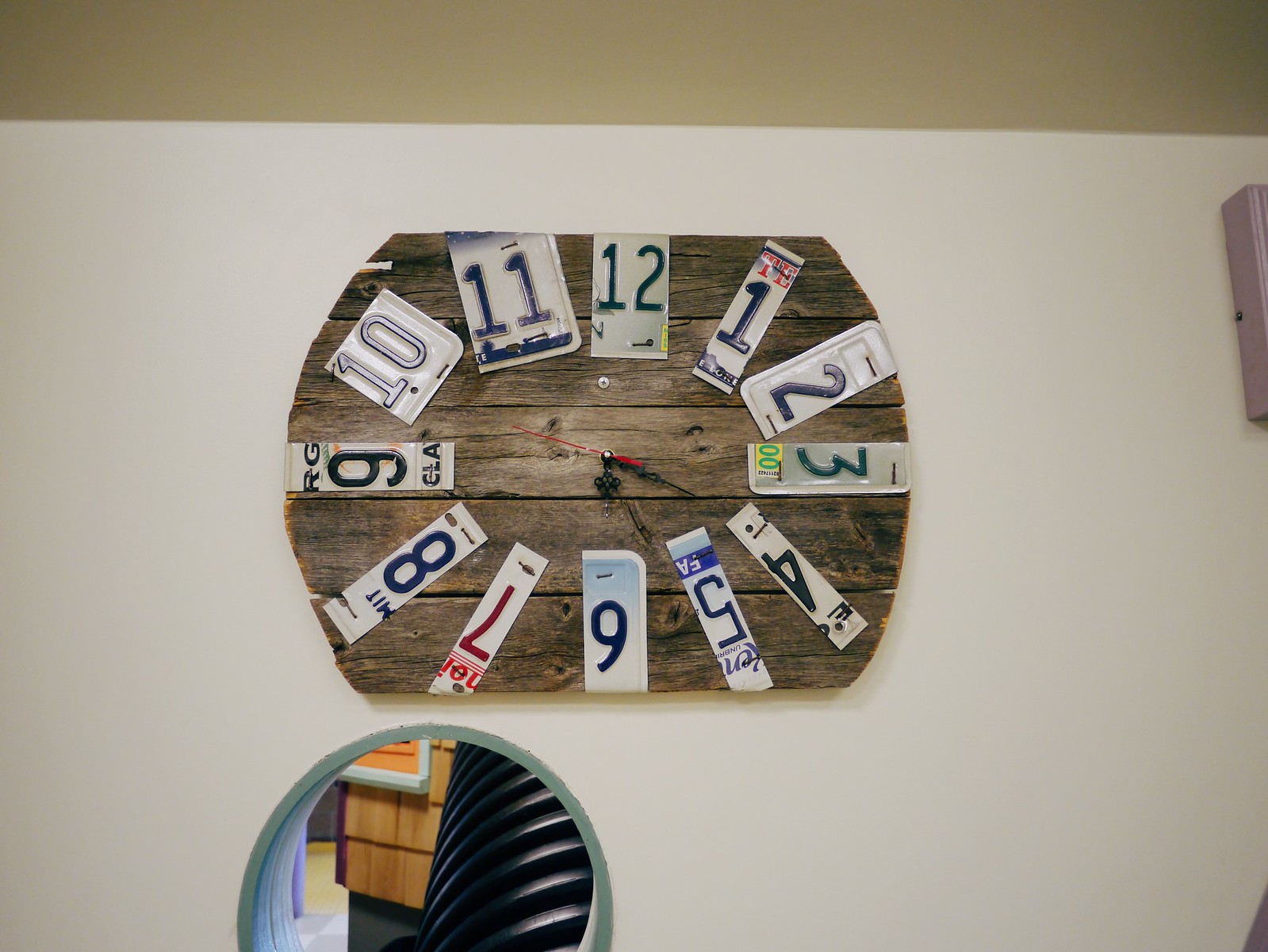This photograph captures a uniquely handcrafted clock hanging on a pristine, white-painted wall. The ceiling, partially visible at the top of the frame, exhibits a rich, gold or dark brown hue, adding a touch of warmth to the scene. Dominating the image is the clock, crafted meticulously from several planks of dark brown wood, showcasing its rustic charm. The clock’s numbers are ingeniously fashioned from pieces of cut-up license plates, displaying an eclectic mix of colors and textures. The numbers 12, 1, 2, 3, 4, and so forth encircle the clock, which has an unusual shape—almost circular but with flat sections at the top and bottom, resembling a rounded rectangle.

The clock is outfitted with black metal hour and minute hands, complemented by a contrasting red metal second hand, all pointing towards various times in a dynamic pose. At the bottom left, near the center, a mirrored segment reflects part of the room. In the reflection, a black, ridged, segmented piece, possibly a plastic plumbing pipe, can be discerned, adding another layer of intrigue to the scene. The image seamlessly blends elements of craftsmanship, creativity, and industrial aesthetics, making the clock a captivating focal point.